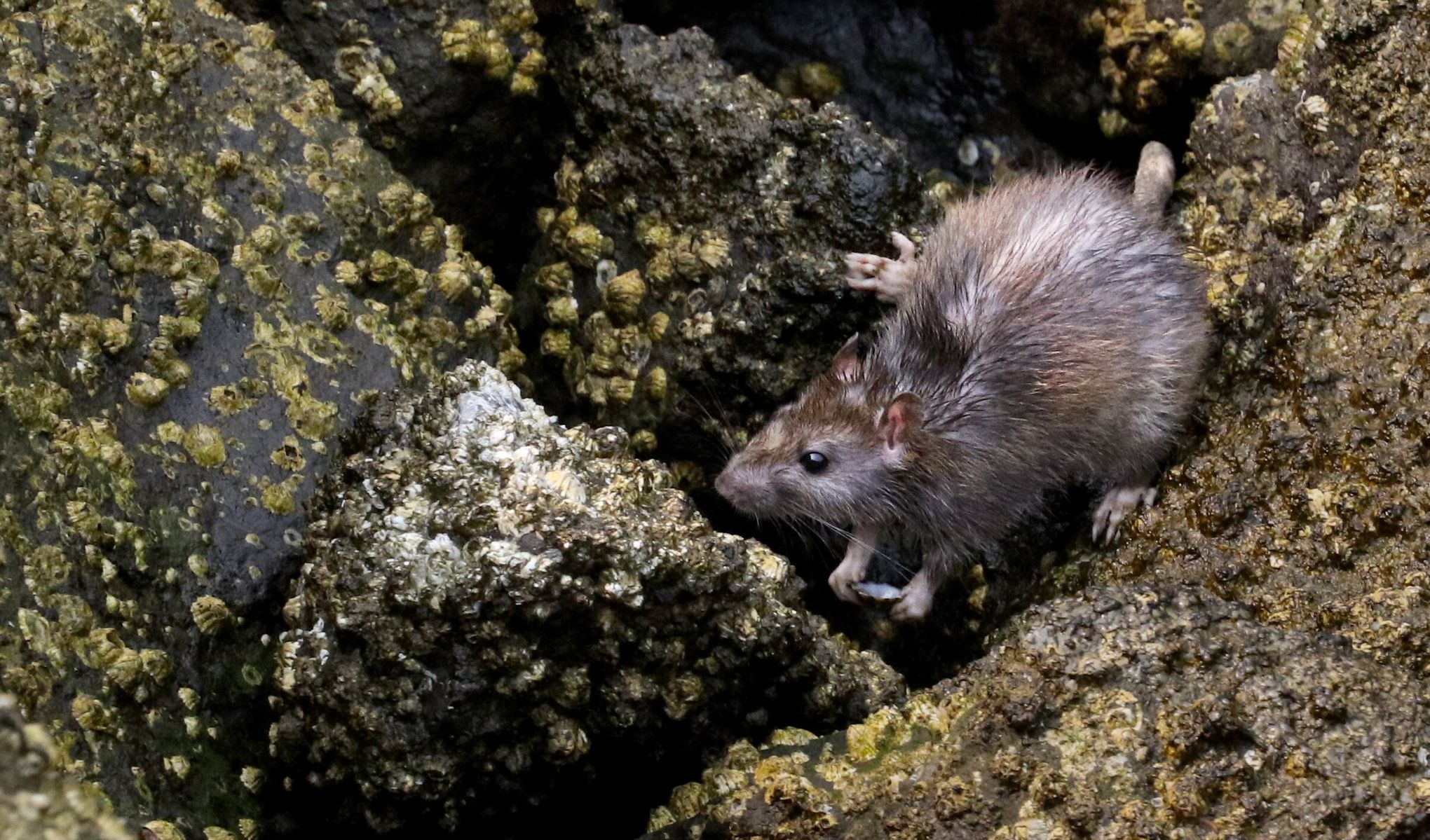In this detailed image, a mouse, adorned with shades of brown, white, and light gray, is nestled between several rocks. The rocks are encrusted with barnacles, mussels, and vibrant mosses in hues of yellow and light green, indicating their proximity to the ocean or a wet area. The mouse appears to be drying off, possibly from a recent dip in the water, as it holds a mussel shell in its paws, much like a human hand. With its thin, damp fur, it looks directly up at the camera capturing an almost intimate moment. Its tan tail, speckled with black, and hand-like back feet are also visible, adding to the intricate details of the scene. The rocky surroundings, paired with the mouse's intense gaze, create a captivating snapshot of oceanic wildlife.